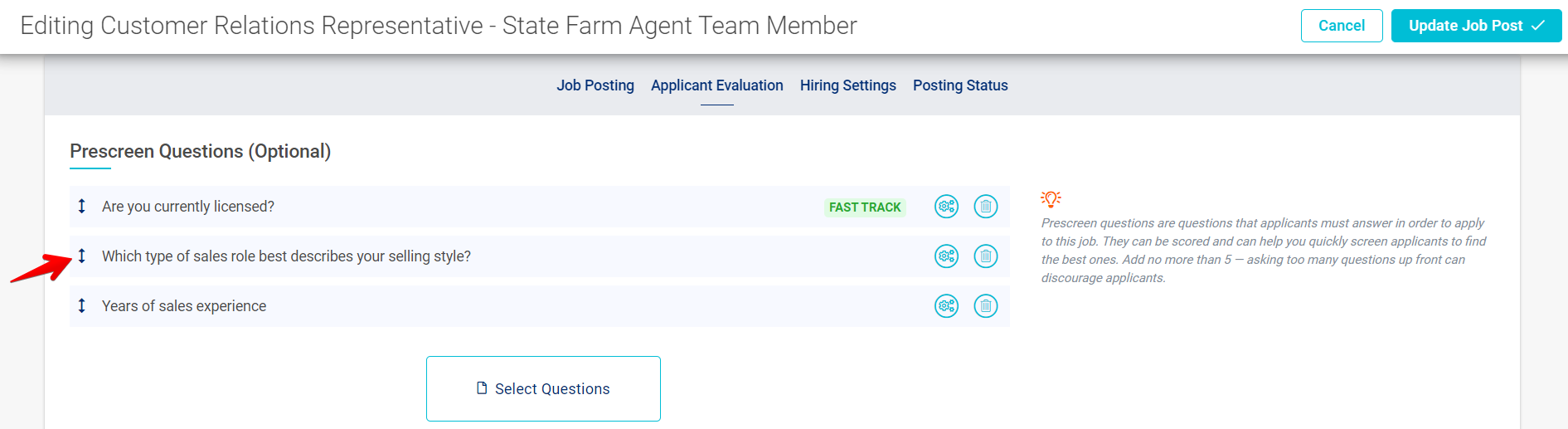The image depicts a screenshot from a computer interface related to editing a job posting for a Customer Relations Representative under the title "State Farm Agent Team Member." At the top of the screen, there are two clickable buttons on the far right: a teal "Cancel" button and a teal "Update Job Post" button with white text and a checkmark.

Below this header, there is a gray inset area featuring dropdown menus labeled "Job Posting," "Applicant Evaluation," "Hiring Settings," and "Posting Status." Moving further down, there is a section titled "Pre-Screen Questions" followed by the word "Optional" in parentheses.

This pre-screen section includes three specific questions:
1. "Are you currently licensed?"
2. "Which type of sales role best describes your selling style?" 
3. "Years of sales experience."

A red arrow has been digitally added to the screen, pointing towards the second question about the applicant's selling style.